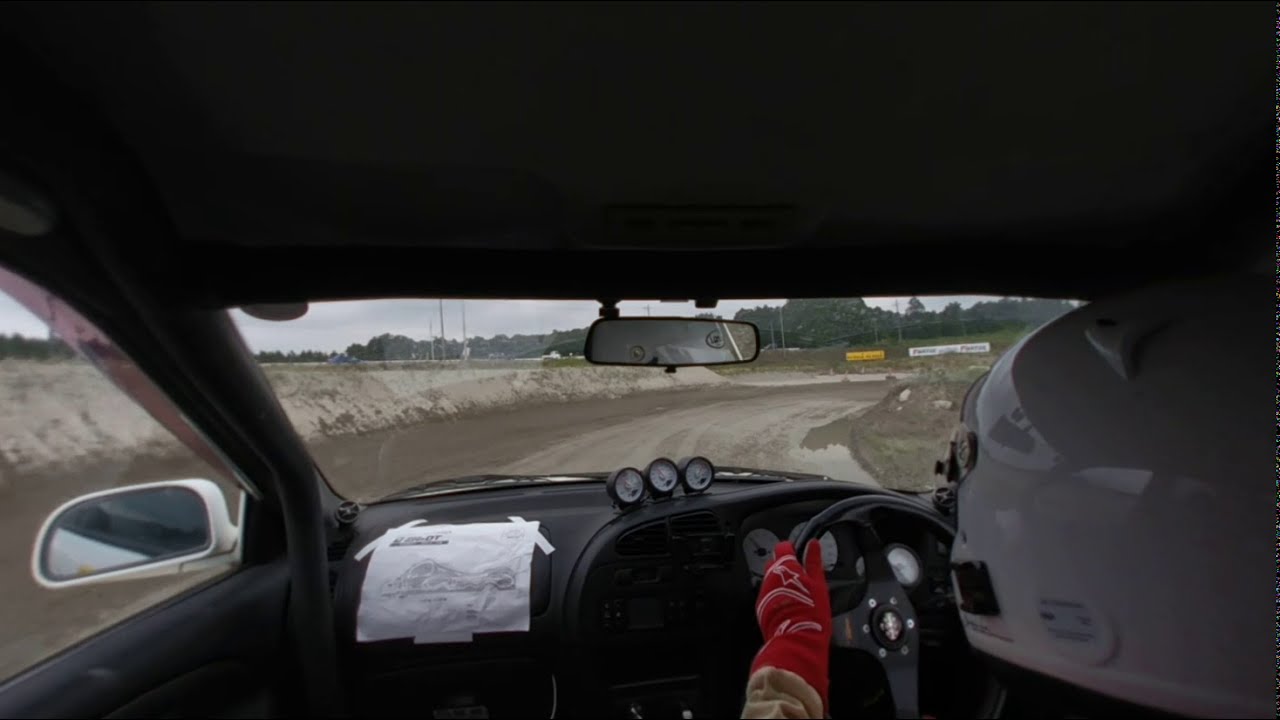The image captures a point-of-view shot from inside a race car, presumably from the backseat angle. The driver is prominently featured, wearing a semi-glossy white helmet with a clear visor and red gloves adorned with white piping. The driver's gloved hands are gripping a black steering wheel, which is turned to the right. Ahead of them lies a dirt track, notably wet and muddy, curving toward the right. The vehicle’s interior is dark, either black or dark gray, with a completely black dashboard. Three gauges with white faces and black numbers are visible, along with a piece of white paper taped to the left side of the dashboard. Outside, the scene reveals a brown dirt path, with a steep dirt slope to the left and brown patches of dirt to the right. Distant yellow and white signs loom on the track, hinting at upcoming turns. The overall environment appears gloomy, with no direct sunlight visible, suggesting overcast weather. This race car, suggested by its speed and specialized interior (including a rain guard), is a white vehicle, as glimpsed through the side view mirror.